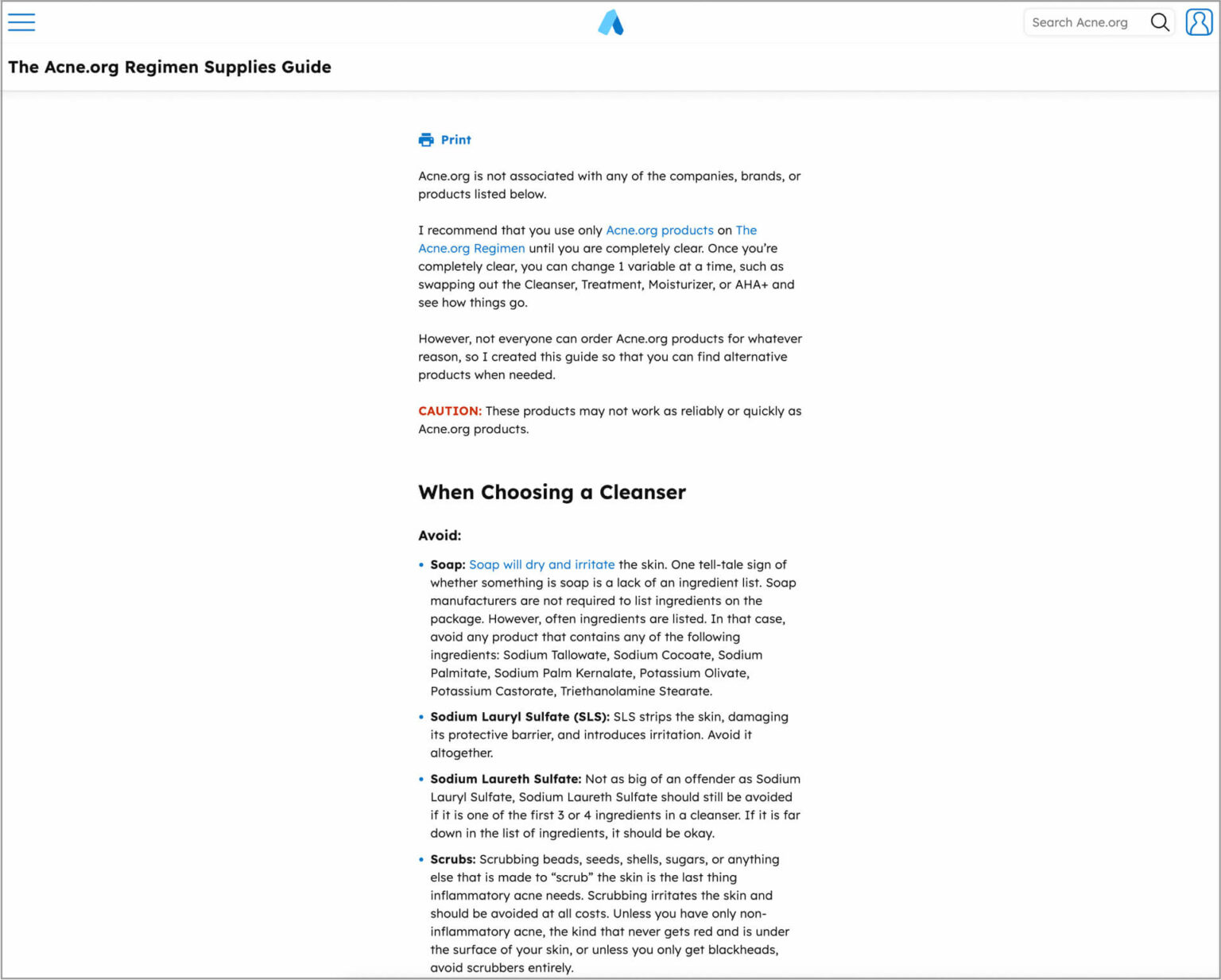This is a detailed screenshot from the Acne.org Regimen Supplies Guide web page. At the top center of the header, there's the Acne symbol, representing Acne.com. The header also features the title "The Acne.org Regimen Supplies Guide" on the top left side. On the top right, there is a search bar alongside a silhouette icon for the user profile.

The main body of the web page showcases a clean design with a white background and black text. At the very top, there's a print icon followed by the word "Print" in blue. Directly below, a disclaimer reads: "Acne.org is not associated with any of the companies, brands, or products listed below." Additionally, there's a caution advising that "these products may not work as reliably or as quickly as Acne.org products."

In the second section, titled "When Choosing a Cleanser," one of the points is to avoid soap, highlighted by the statement "soap will dry and irritate the skin," where "soap will dry and irritate" is emphasized in blue text. It further adds that one telltale sign of a product being soap is the absence of an ingredient list.